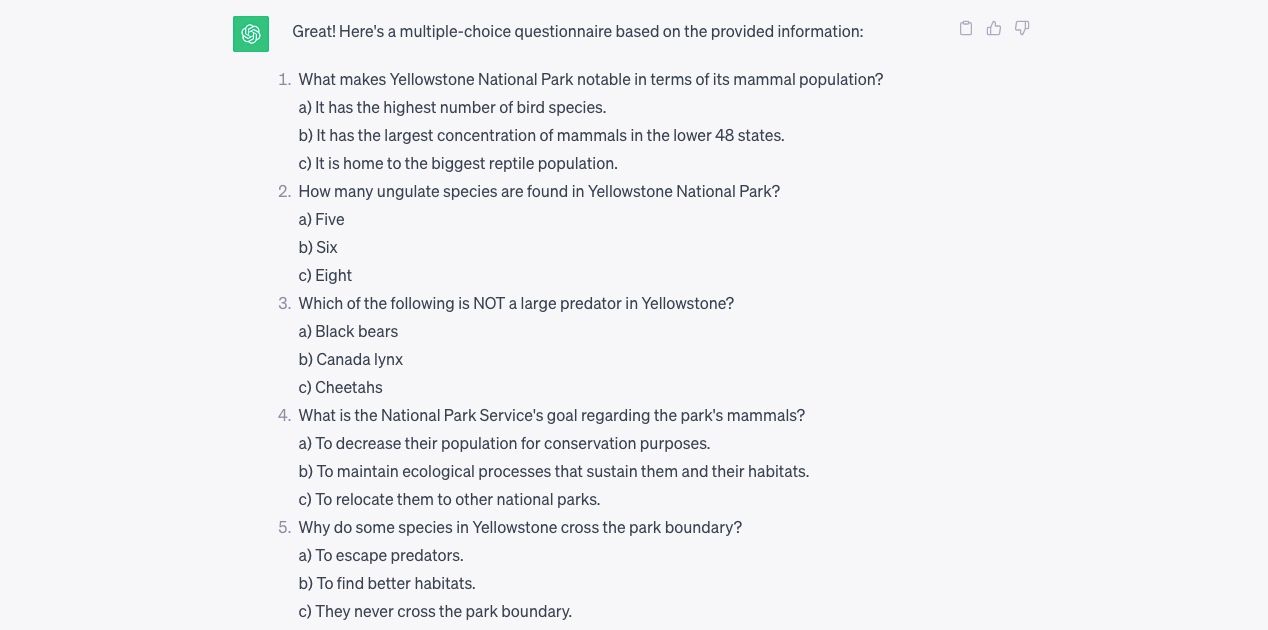This is a rectangular online image, approximately one and two-thirds times wider than it is high. It features a quiz set against a light gray background with no border. Thick margins, accounting for about 20% of the width on both sides, frame the central content.

In the upper left area of the central section, just right of the left margin, there is a green square displaying a white abstract hexagonal or octagonal shape. To the right of this green square, dark gray text reads: "Great! Here's a multiple-choice questionnaire based on the provided information:" Following this are three light gray icons: a thumbs-up icon in the middle, a thumbs-down icon on the right, and a clipboard icon on the left.

Beneath this heading are five questions, each numbered 1 to 5 with periods following the numbers. Each question offers three possible answer choices labeled A, B, and C, each followed by a parenthesis. 

1. The first question asks, "What makes Yellowstone National Park notable in terms of its mammal population?" The answer choices are:
   - A. It has the highest number of bird species.
   - B. It has the highest concentration of mammals in the lower 48 states.
   - C. It is home to the biggest reptile population.

2. The second question is, "How many ungulate species are found in Yellowstone National Park?" The answer choices are:
   - A. Five.
   - B. Six.
   - C. Eight.

3. The third question asks, "Which of the following is NOT a large predator in Yellowstone?" The word "NOT" appears in all capital letters for emphasis. The answer choices are:
   - A. Black bears.
   - B. Canadian lynx.
   - C. Cheetahs.

4. The fourth question reads, "What is the National Park Service's goal regarding the park's mammals?" The answer choices are:
   - A. To decrease their population for conservation purposes.
   - B. To maintain ecological processes that sustain them and their habitats.
   - C. To relocate them to other national parks.

5. The fifth question, which appears to be partially cut off and might continue if the page is scrolled down, asks, "Why do some species in Yellowstone cross the park boundary?" The answer choices are:
   - A. To escape predators.
   - B. To find better habitats.
   - C. They never cross the park boundary.

Each answer choice ends with a period. The image seems to represent part of an interactive quiz about Yellowstone National Park's wildlife and conservation efforts.